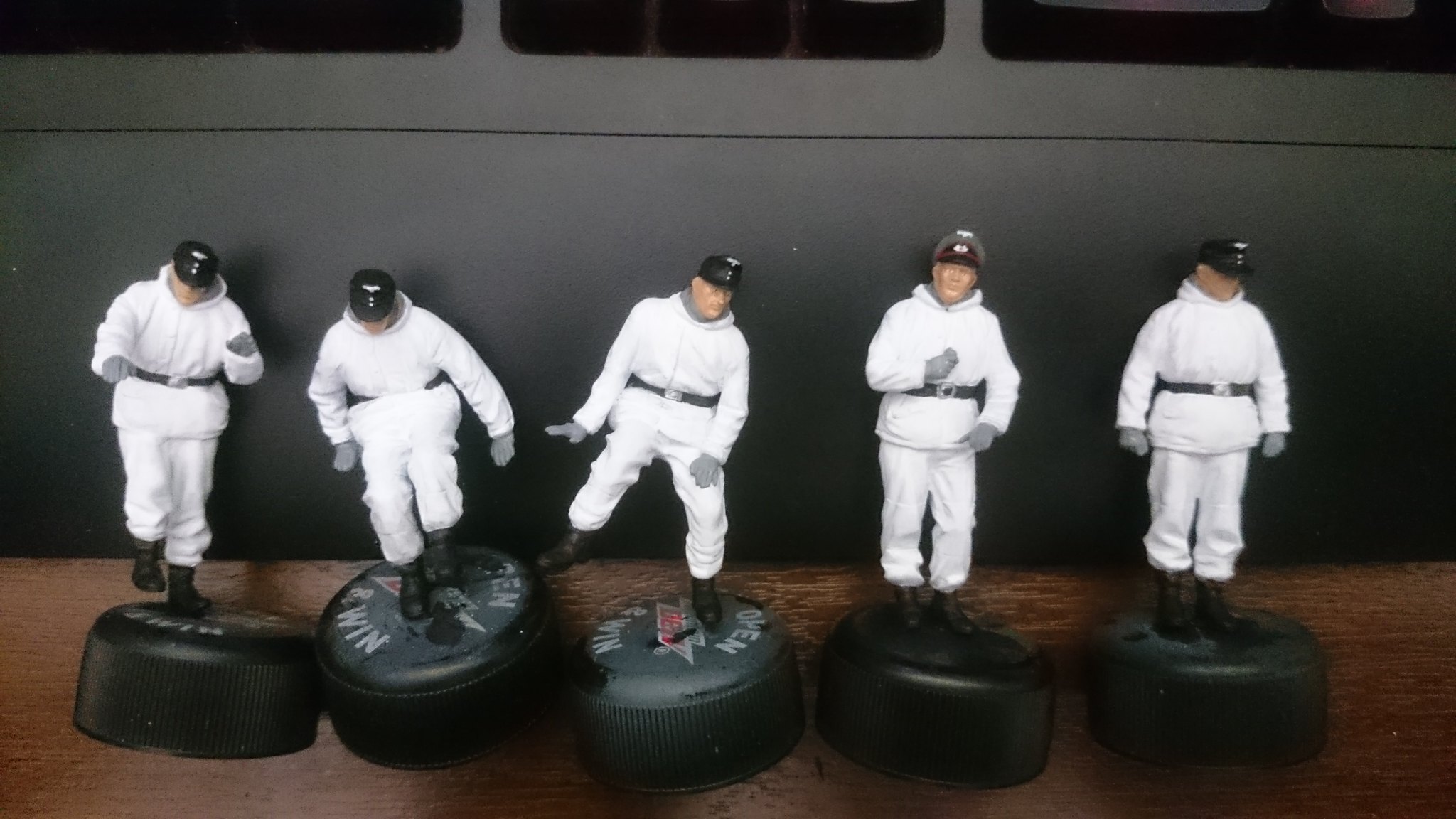The photograph displays a meticulously arranged scene featuring five male action figures dressed in white winter military outfits standing upright on dark green bottle caps, possibly old Mountain Dew twist-offs, which resemble thick hockey pucks. These figures, which have light skin, are adorned in detailed uniforms that include white coats with black belts, white pants, and black leather boots. Each figure also wears a military-type hat resembling a baseball cap with small gold insignias, contributing to their cohesive look. They stand on a dark wooden table that transitions from brown at the bottom to gray towards the viewer's eye, adding a rich layer of depth and color variation. Behind the figures is a backdrop of a dark gray wall, adorned at the top with the bottom halves of windows, distinguished by thin black lines and lighter shades of gray in the center. Balancing on their rounded, slightly poofy tops, the bottle caps provide an uneven yet stable platform for the figures, some of which tilt slightly to the left or right. Overall, the detailed setting and carefully posed figures suggest a deliberate and artistic composition.